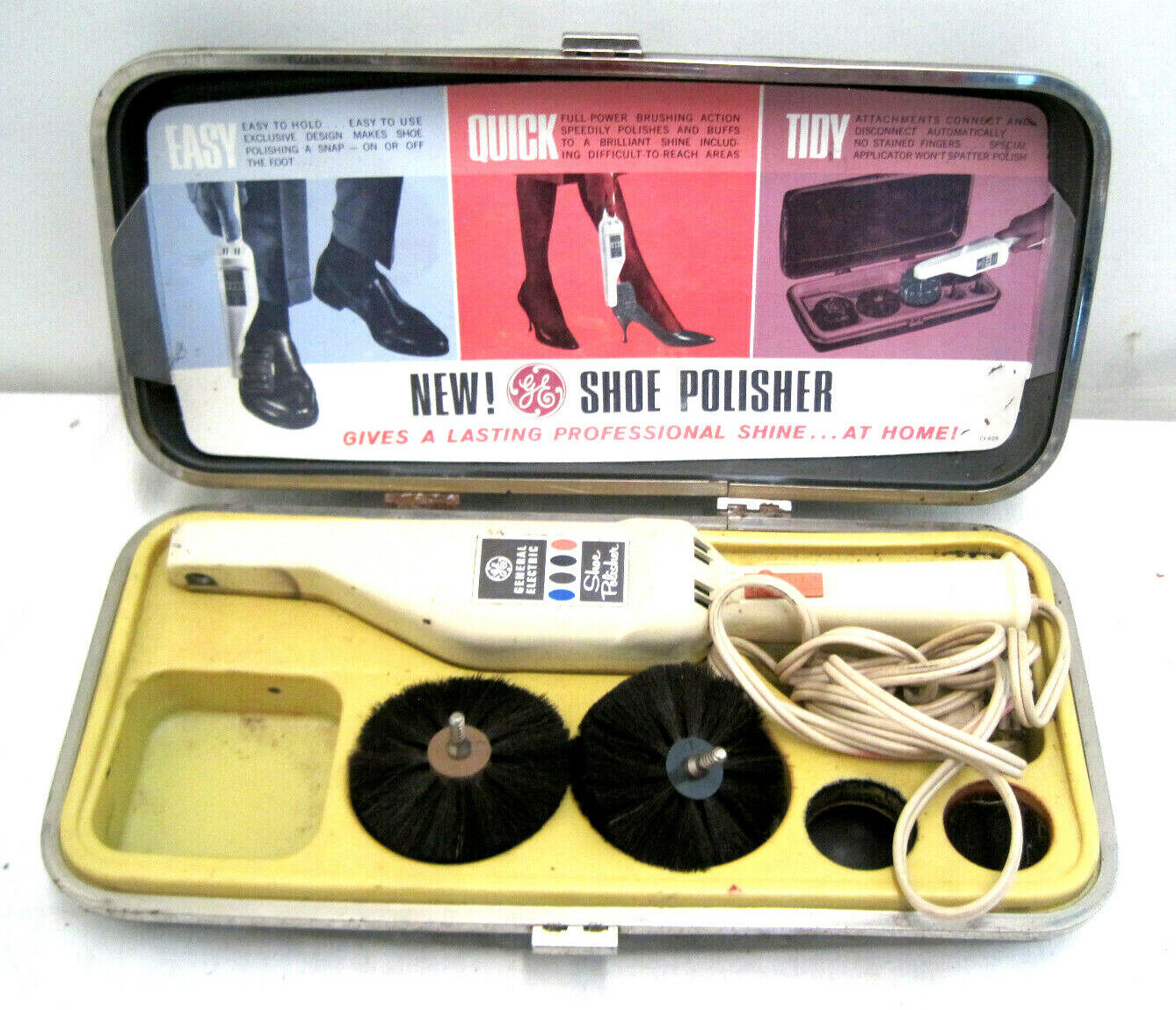This photograph depicts an antique-looking shoe polisher, likely from the 1960s, displayed on a white shelf with an off-white background. The open case, resembling an old-school clamshell suitcase trimmed in silver metal, showcases a "new GE shoe polisher". The top inside of the case features a cardboard display with segments titled "Easy," "Quick," and "Tidy." 

In the "Easy" section, marked in white font on a blue background, the instructions highlight its ease of use and exclusive design, demonstrating a man polishing his black shoes with the device. The "Quick" section, in white font on a pink background, emphasizes the appliance's full power brushing action, showcased by a woman using it on her high heels. The "Tidy" segment, in purple, notes the ease of attaching and detaching brushes and shows a picture of the shoe polishing kit.

The bottom inside of the case is banana yellow and contains compartments holding the parts of the polisher: two large round brushes, a white handheld wand with an orange switch, and a coiled white extension cord. Despite its age and apparent dirt marks, the kit remains intact, offering a glimpse into mid-century home appliance design and functionality.